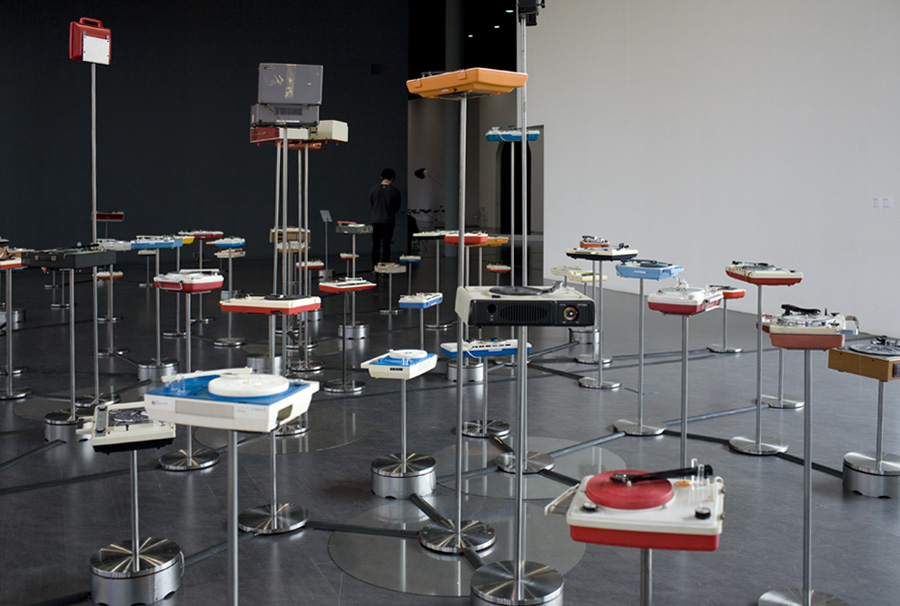The photo captures an exhibition of approximately 50-60 vintage, toy-like record players displayed in a large indoor space with very high ceilings. The room features a dark grey left wall, a white right wall, and a lighter grey floor. The record players, designed to play large black vinyl records, sit mounted on silver, stainless steel stands of varying heights, each anchored by circular metallic bases. The bases and stands connect via interlinking stainless steel or chrome components. Dominantly colored in red and white, there are also blue and white, yellow and white, orange and white, and brown and white record players scattered throughout the room. Some record players are mounted on taller poles, while others are closer to the ground. The display is arranged almost symmetrically, giving it an organized yet diverse appearance. The overall impression is of a whimsical yet nostalgic collection, evoking a sense of playful past eras.